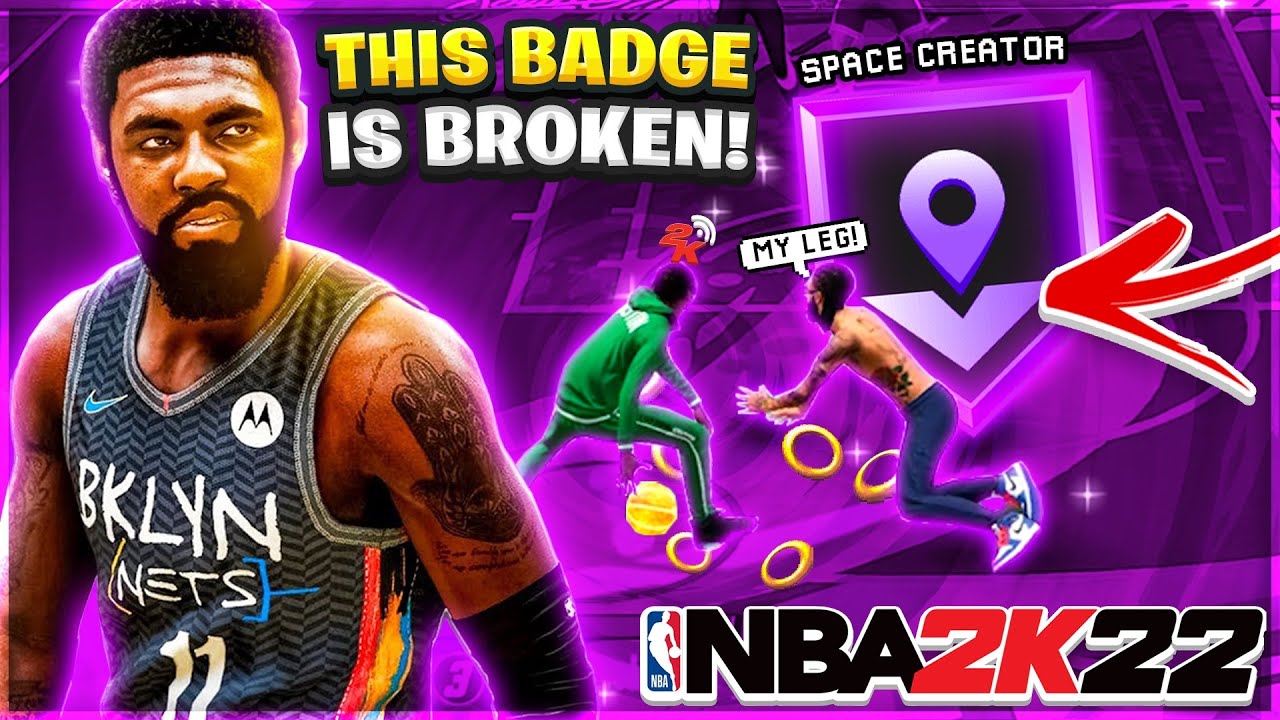In the image, a man is prominently featured against a predominantly purple background, likely set on a basketball court. He is wearing a jersey with "BKLYN" and "Nike" logos, along with several sponsorships including "Boterola." The jersey has the number 11 on it. The man has a notable tattoo of a hand with an eye on his shoulder and is wearing a compression sleeve on one of his arms. He has a thick beard, noticeable wrinkles on his forehead, and is of short stature. 

Text on the image includes various phrases: "This Badge" is written at the top, "It's Broken" is displayed in yellow text at his waist, and "Space Creator" is also visible. Purple pins with a red arrow point towards unknown elements in the scene. On the far right, a person in a green hoodie is identified by the text "about 2K wavy." Additional graphical elements include exclamations such as "boom, boom, boom" and the phrase "My Leg" near someone wearing blue pants, Nike shoes, and gold rings. 

The setting is filled with vibrant details like stars in the bottom right corner and the text "NBA 2K22." There is also a reflection on the man's forehead, signifying sweat on the left side. Additional text appears both above and below the tattoo on his shoulder, although it is not fully detailed in the description.